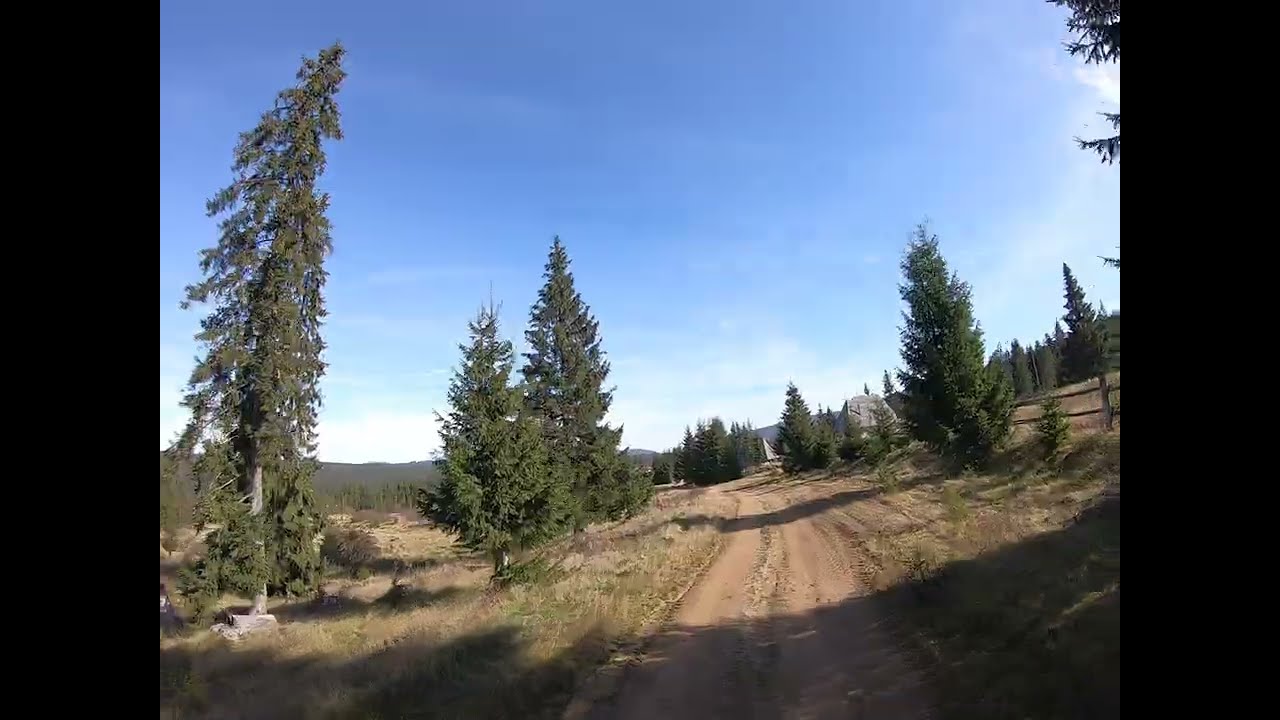This image, likely taken from a GoPro or dashcam with a fisheye effect, captures a sunlit dirt road flanked by thinly spaced evergreen trees, probably somewhere in the mountain west of the United States. The road, brown with a strip of grass running through its middle, seems wide enough to accommodate vehicles on either side. The sky above is a vivid blue with a few wispy white clouds, gradually lightening toward the horizon where it meets the trees. On the right side of the road, a wooden fence with vertical and horizontal poles extends into the distance. To the left, the trees include a very tall one that appears to lean slightly due to the camera's bending perspective, while two smaller trees stand straighter yet maintain a slight tilt. The scene hints at mountainous terrain in the distance, suggesting the road cuts through a scenic, lightly forested area.